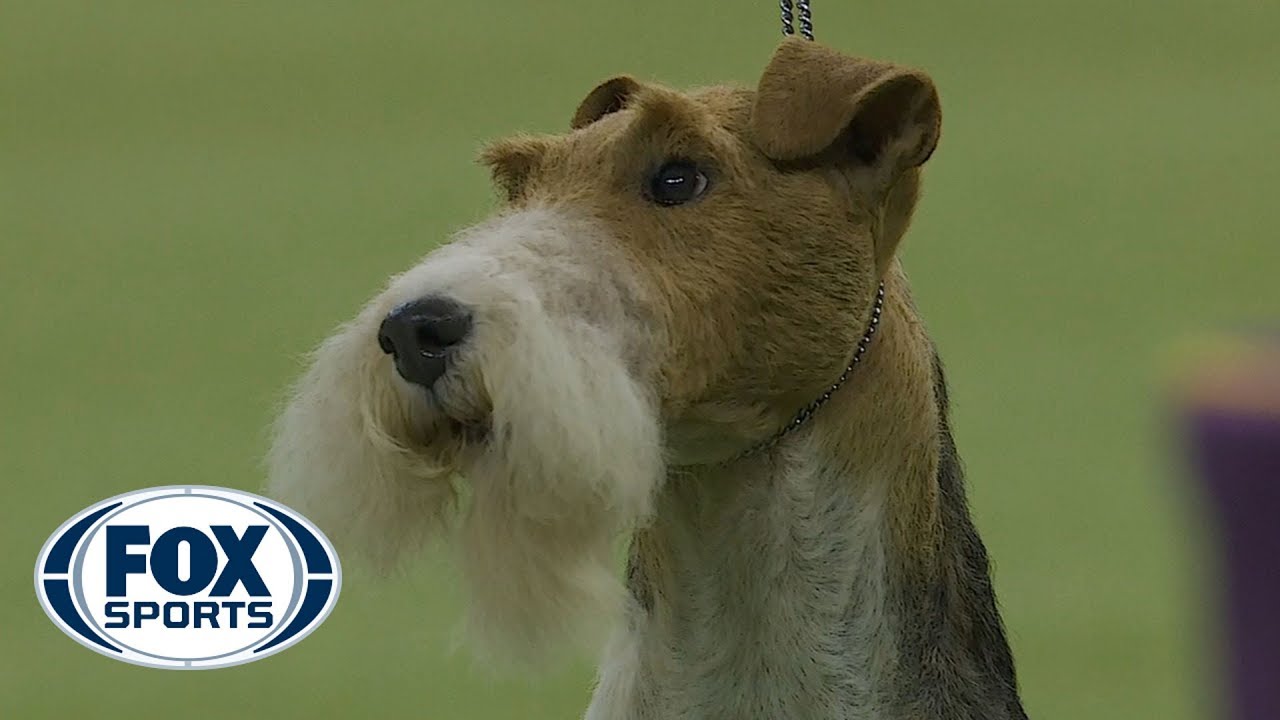In this detailed image taken at a dog show, the focus is a terrier-type dog, possibly a Schnauzer, facing its handler with a proud and attentive expression. The dog’s characteristic features include a long snout adorned with a distinctive off-white beard and mustache, set off by its mostly brown fur. Notable off-white patches are visible around the dog's face, on its chest, and under the long neck. The dog's ears fold forward endearingly over its head. The background is a green screen, effectively highlighting the dog and making its detailed features stand out crisply. In the lower left-hand corner, the Fox Sports emblem is noticeable, with its semicircle shape and large blue "Fox Sports" lettering. The emblem has blue highlights that add to the overall polished composition of the photograph, where the dog's impressive grooming and the neatness of the image are prominently showcased.